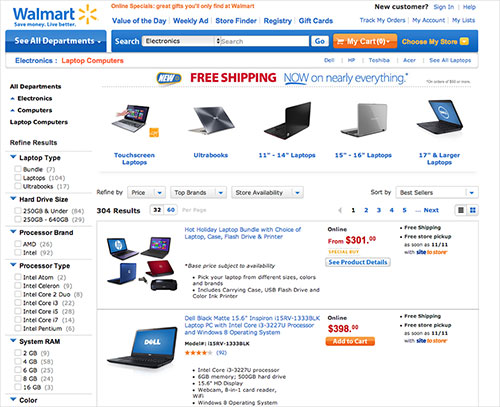The image displays a comprehensive Walmart web page filled with various features and sections. In the upper left corner, there is a prominent Walmart advertisement, featuring the iconic yellow sunburst logo alongside the Walmart name in blue. The ad promotes "Online Specials of Great Gifts You'll Only Find at Walmart," highlighted in orange at the top of the page.

Directly below the ad, a navigation bar offers quick links labeled "Value of the Day," "Weekly Ad," "Store Finder," "Registry," and "Gift Cards." On the right side of the page, options for customer engagement are listed, including "New Customer" in black text, as well as links for "Sign In," "Help," "Track Orders," "My Account," and "My List."

A blue search bar dominates the center, with the default search category set to "Electronics." Adjacent to the search bar, an orange rectangle labeled "My Cart" currently indicates zero items. There is also a drop-down menu from which users can choose their preferred store location.

The main content showcases a variety of electronics for sale, categorized under departments such as "Electronics," "Computers," and specifically "Laptops." Users can refine their search results by selecting specific criteria like "Laptop Type," "Hard Drive Size," "Processor Brand," "Processor Type," "System RAM," and even "Color."

Highlighted prominently are two featured laptops, each within its own box. These boxes display an image of the laptop, a brief description, and the price, emphasized in red. Additional labels include "Free Shipping" in red text and "New," outlined in yellow, emphasizing the freshness of the offers. The webpage also shows a variety of other laptop images below the main highlighted choices, providing an extensive selection for potential buyers.